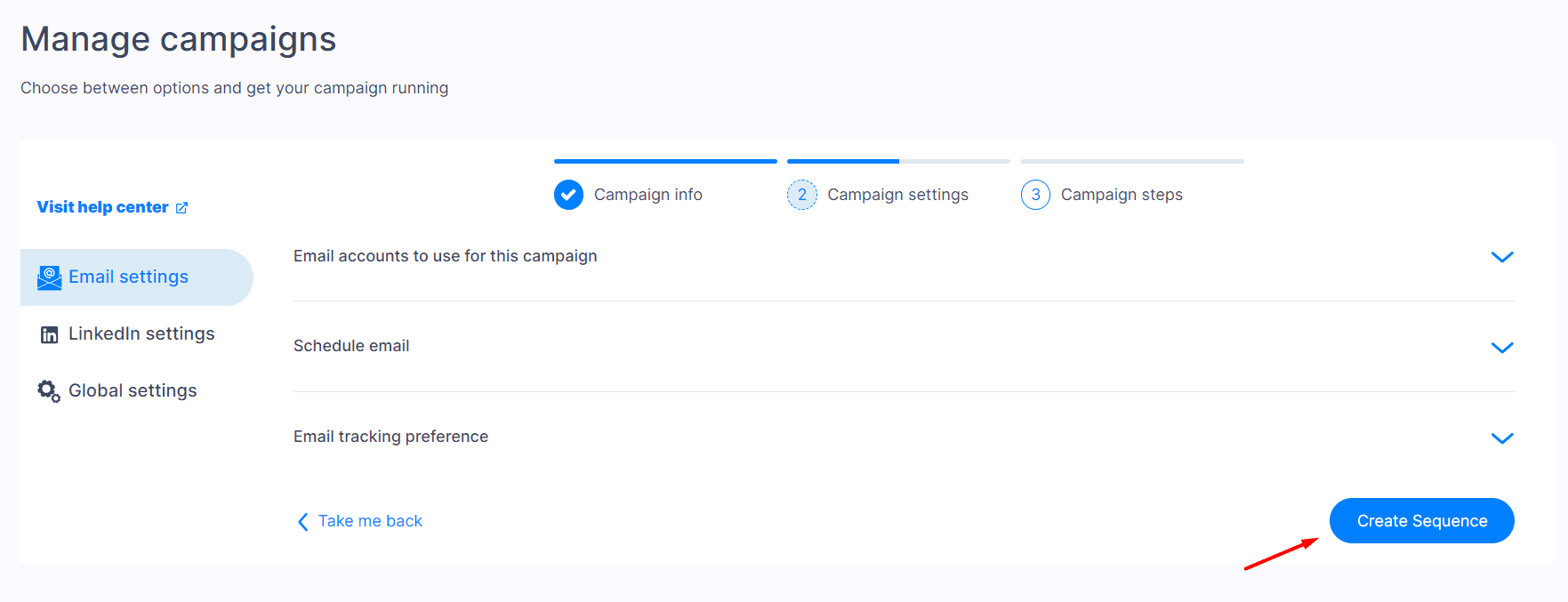The screenshot displays an interface of an email campaign management software. The interface showcases various options for managing email campaigns. On the left sidebar, there are tabs listed as Email Settings, LinkedIn, Global Settings, Email Accounts Used for This, Schedule Email, and Email Tracking. In the center of the screen, a blue, pill-shaped button labeled "Create Sequence" is highlighted by a red arrow pointing towards it. Surrounding this button are several dropdown menus, indicating customizable options for user interactions. The design is predominantly light gray with a white background, while interactive buttons and elements are accentuated in a sky-blue color for better visibility and user experience.